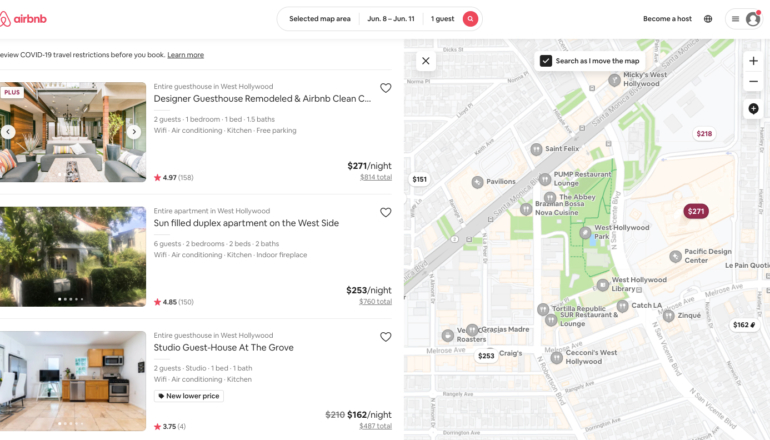This screenshot from Airbnb showcases a selection of accommodations in West Hollywood for one guest, with travel dates from June 8 to June 11.

At the top, the familiar Airbnb logo appears in lowercase red letters. Below, the prompt "Become a host" is displayed alongside a reminder to review COVID-19 travel restrictions before booking, with a link to learn more.

On the left side, there is a photograph of a spacious, airy room featuring gray couches. This is part of an "Entire guest house in West Hollywood," which is listed as a "Designer guest house remodeled to Airbnb Clean standards." It accommodates two guests with one bedroom, one bed, and 1.5 baths. Amenities include Wi-Fi, air conditioning, a kitchen, and free parking. The property has received an average rating of 4.97 stars from 158 reviews and is priced at $271 per night, totaling $814 for the stay.

Adjacent to that, a photo depicts a house surrounded by tall green trees and lush shrubbery. This is for an "Entire apartment in West Hollywood" described as a "Sun-drenched duplex apartment on the west side." Suitable for six guests, it features two bedrooms, two beds, and two baths. Additional amenities include Wi-Fi, air conditioning, a kitchen, and an indoor fireplace. It boasts an average rating of 4.85 stars from 150 reviews and is available for $253 per night, totaling $760.

Next, there's an image showcasing a small kitchen area equipped with wooden cabinets and stainless steel appliances. To the left, a TV sits on a pedestal, and part of a dining room table and chairs are visible at the far left of the image. The floor is polished, giving the room a tidy appearance. This listing is for an "Entire guest house in West Hollywood" titled "Studio guest house at the Grove." Accommodating two guests, it offers a studio layout with one bed and one bath. The amenities include Wi-Fi, air conditioning, and a kitchen. The property, which has recently been reduced in price, now costs $162 per night (down from $210), totaling $487. It holds an average rating of 3.75 stars from 4 reviews.

To the right of these listings, a detailed map highlights various notable locations in West Hollywood, including Pump Restaurant Lounge, The Abbey, Nova Cuisine, Pavilions, West Hollywood Park, West Hollywood Library, Soar Restaurant and Lounge, Tortilla Republic, Cecconi's West Hollywood, Catch LA, Zinc, and the Pacific Design Center.